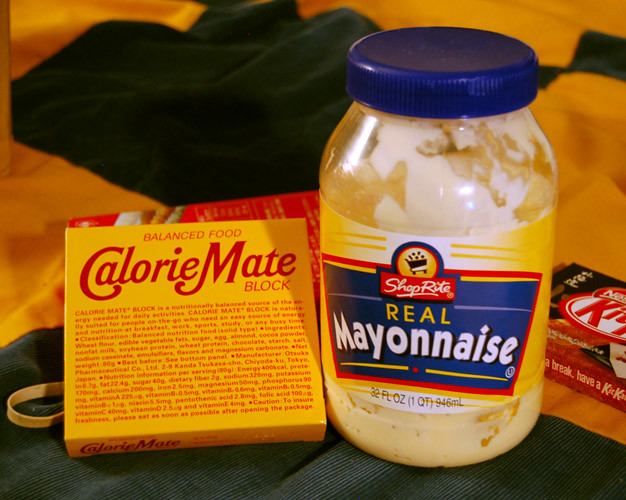This is a square color photograph of three distinct items displayed on a light-colored wooden table. The items are placed on a gray ribbed placemat and have a green, slightly bunched-up cloth as a background. On the left side of the frame, there is a yellow box labeled "Balanced Food Calorie Mate Block" which features red writing. Behind this box, in the lower-left corner, rests a tan elastic band next to an indistinct red box. Next to the Calorie Mate Block is a clear, nearly empty plastic jar of ShopRite Real Mayonnaise featuring a blue screw-on cap and a blue label with red and yellow text. Following the jar, to the far right, is a red-packaged KitKat candy bar pack, easily identified by its distinctive white and red lettering.